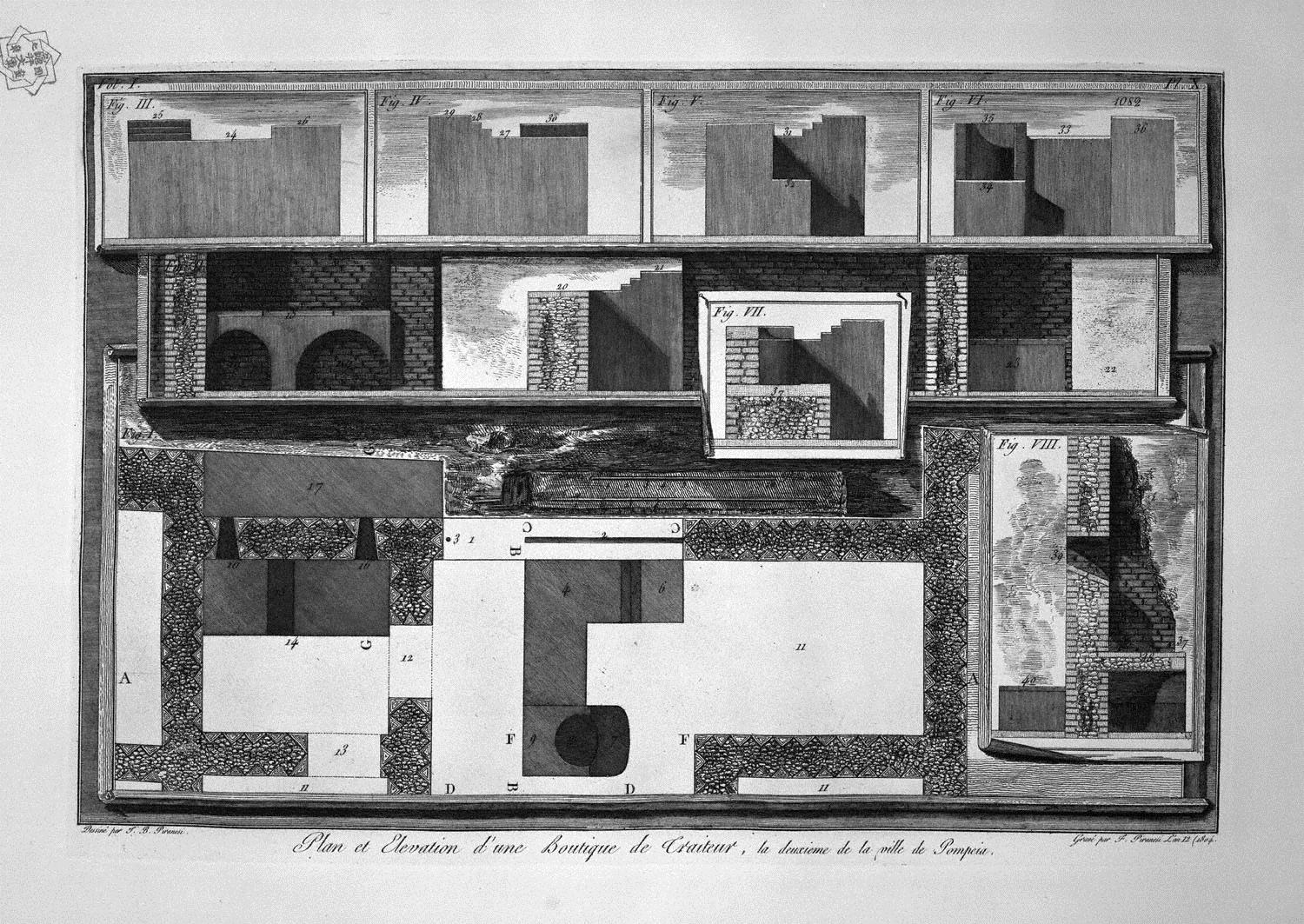The image is a detailed, monochrome architectural drawing, possibly created with charcoal or pencil. It is rendered on a rectangular piece of parchment and displays intricate elements of a building plan, including exterior and interior views, along with top-down layouts. The drawing is labeled in French as "Plan et Elevation d'une Boutique de Créateur," featuring descriptions that are partially legible due to cursive writing and small print. The upper section of the illustration consists of four labeled squares (Fig. 3 to Fig. 6) which depict various exterior sides of a building with block-styled outlines. Below these, there are interior sketches showcasing detailed elements such as inner archways or bridges. Figures 7 and 8 provide further detailed views, including a top-down perspective of courtyards and a depiction of a stairwell. The entire drawing resembles a modern architectural blueprint, complete with numbered areas and labels that suggest a complex, multi-faceted design.